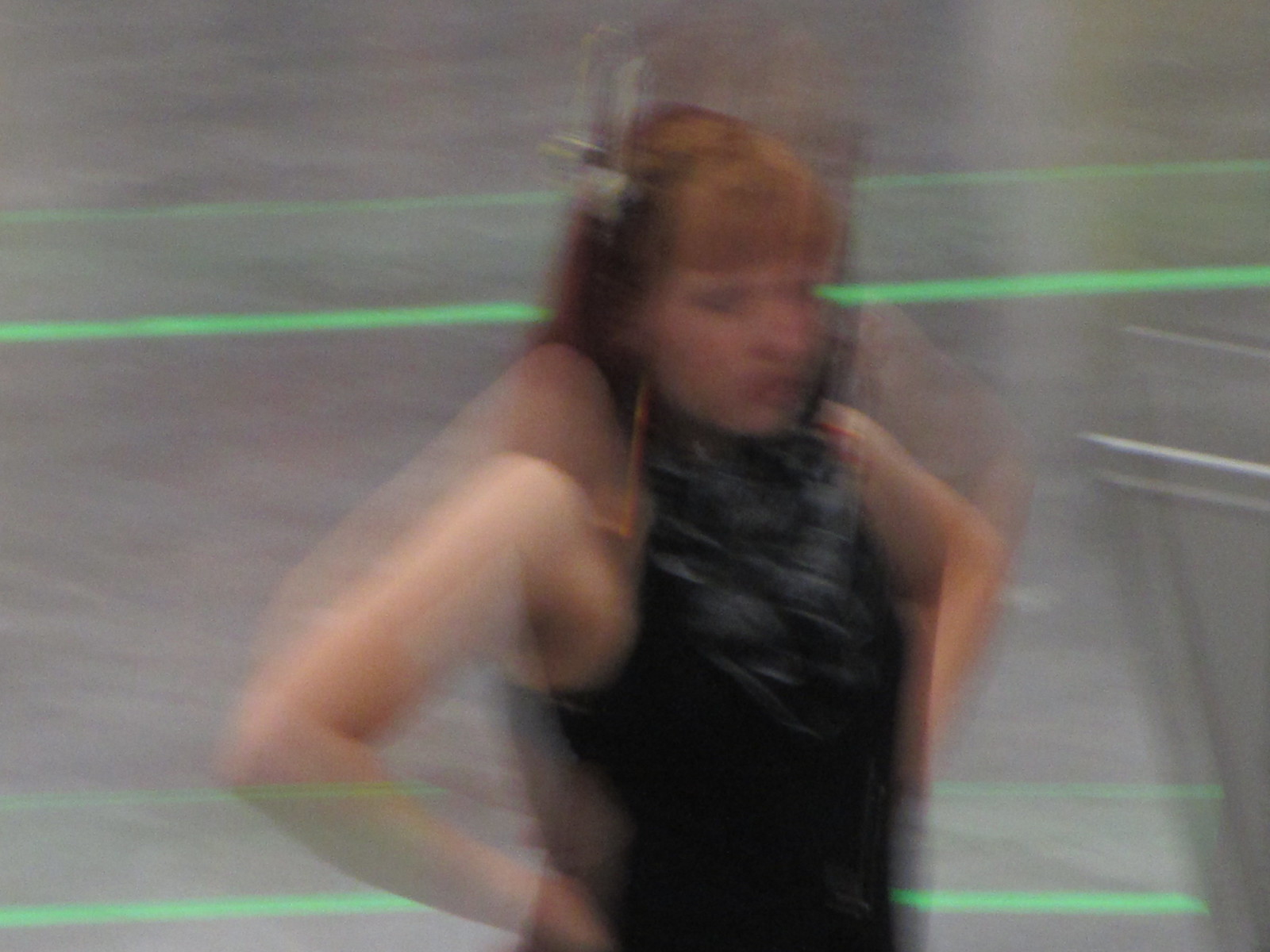A blurry image centers on a woman with short, red hair styled with bangs and a darker red hue down to her shoulders. She accessorizes with a barrette or bow on the left side of her hair. Her skin tone is fair, and while the details are indistinct, the black areas of her eyes, along with the outlines of her nose and mouth, are discernible. She strikes a confident pose with her hands on her hips and her shoulders slightly raised. She wears a sleeveless black top. The background is accentuated by four neon green lines, with two positioned near the top and two near the bottom. Notably, one line cuts behind her hand and arm while another passes behind her elbow, adding an intriguing visual element to the scene.